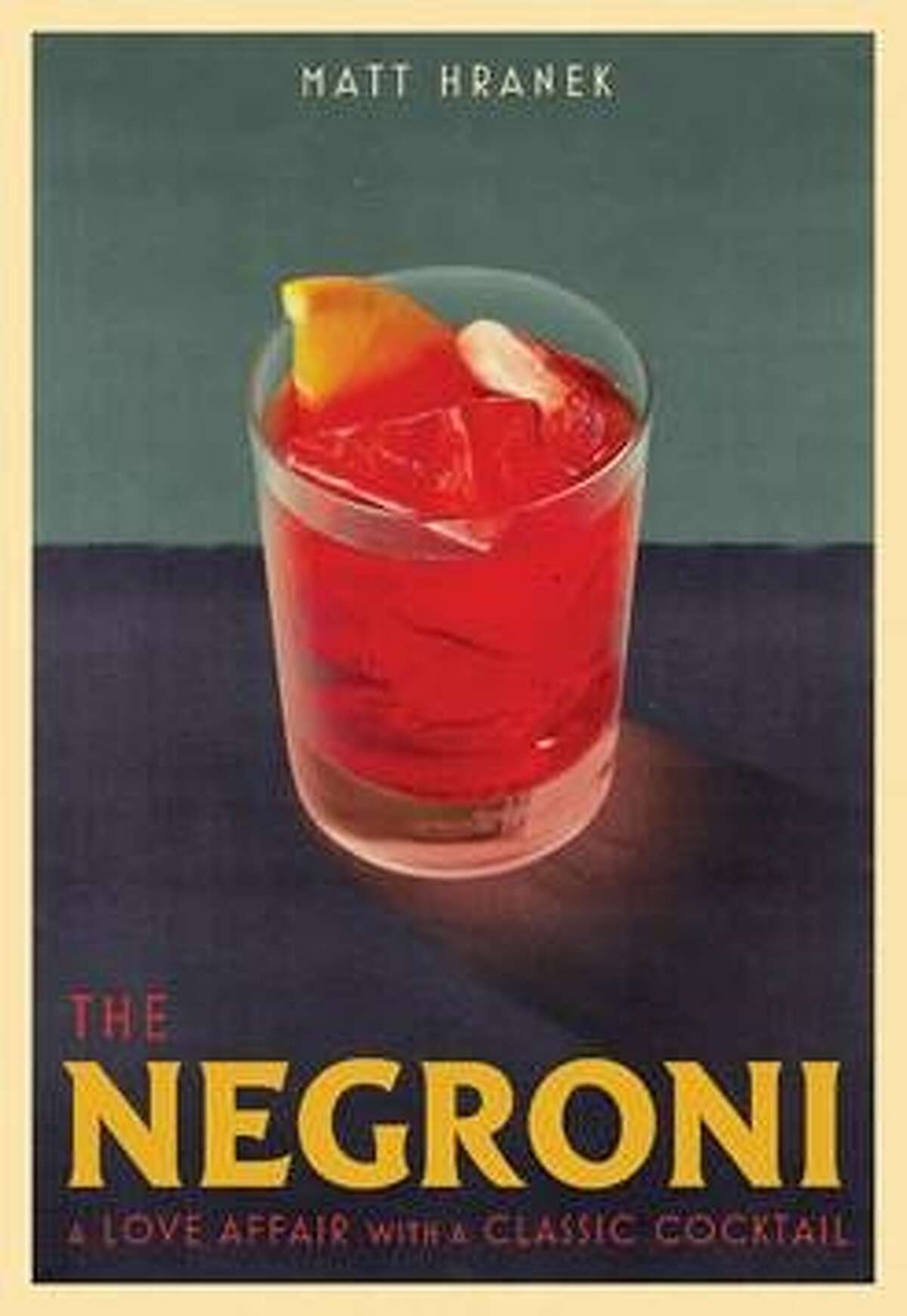The image is a portrait-oriented color photograph cleverly combined with typography to create a poster effect. Centrally framed is a clear glass filled with a vibrant red liquid, identified as a Negroni, garnished with a lemon slice and ice cubes. The glass rests on a dark, nearly black, countertop, while the background features a rich, dark green hue, providing a striking contrast.

At the top of the poster, in small white text, the name "Matt Hranek" is prominently displayed. The lower third of the image is dominated by the text "THE NEGRONI," where "THE" is in red text and "NEGRONI" stands out in bold, gold-colored, all-capital letters. Beneath this, in smaller red lettering, the phrase "a love affair with a classic cocktail" appears, adding an element of poetic allure.

A light gold border surrounds the entire composition, enhancing its classic, vintage poster style. The overall design merges photographic realism with graphic design typography, capturing both the detailed aesthetics of the drink and the elegance of the poster.